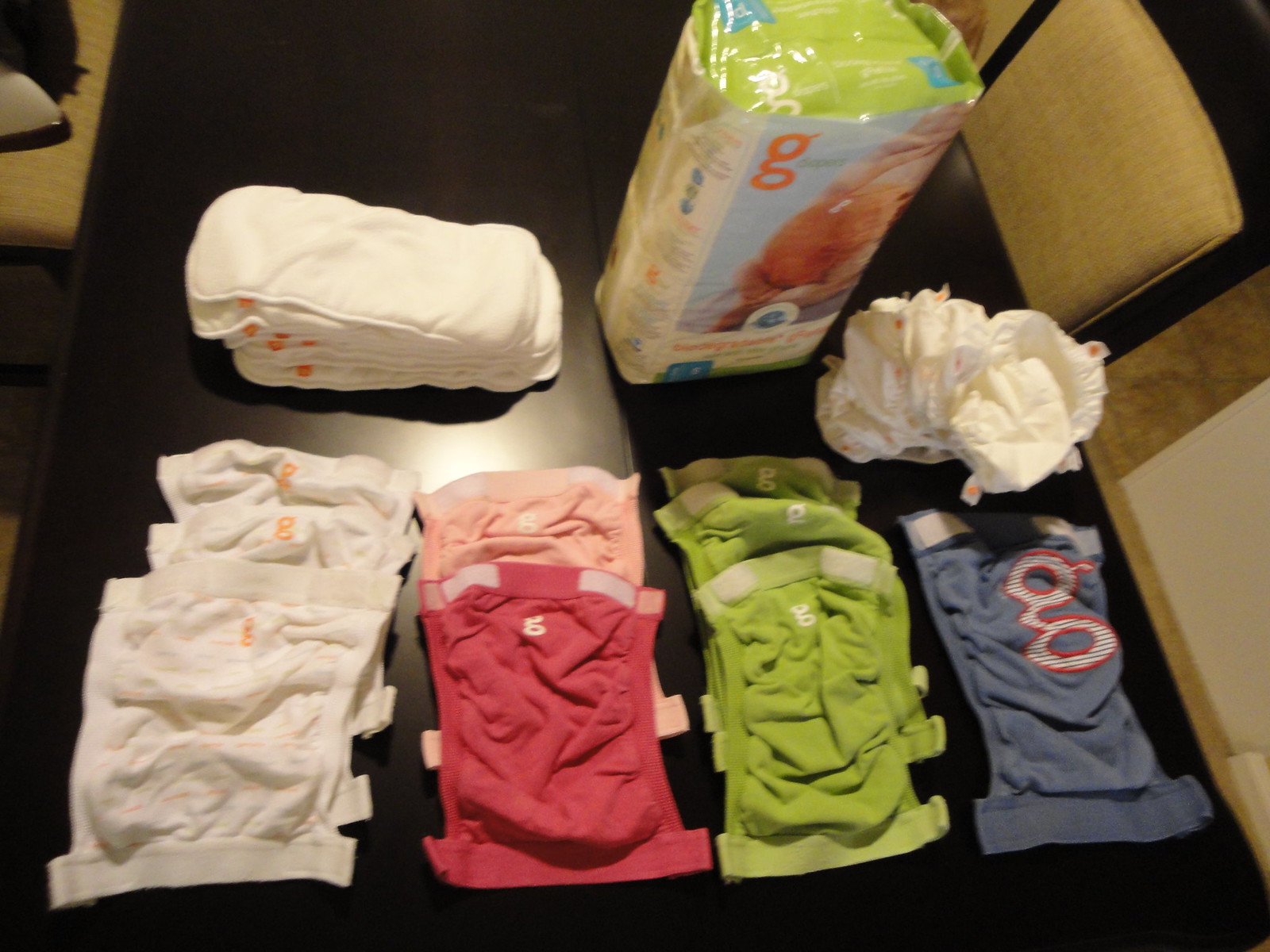In this horizontally oriented color photo, we are looking down at a black dining room table with several piles of washable, reusable baby diapers, neatly lined up by color. The diapers, which are branded with a simple lowercase "g" in cursive, are arranged from left to right. The arrangement starts with three white diapers, followed by two red and salmon-colored ones, next to that are three bright green diapers, and finally, a single bluish denim-colored diaper with a noticeably larger logo. In the background, behind the rows of diapers, there is an unopened packet containing additional light green diapers. The table is flanked by black dining chairs, and an olive green chair is tucked under the table on the left side. The image, likely taken with a phone, captures enough detail to clearly display the organized collection, possibly intended for resale on an online marketplace.